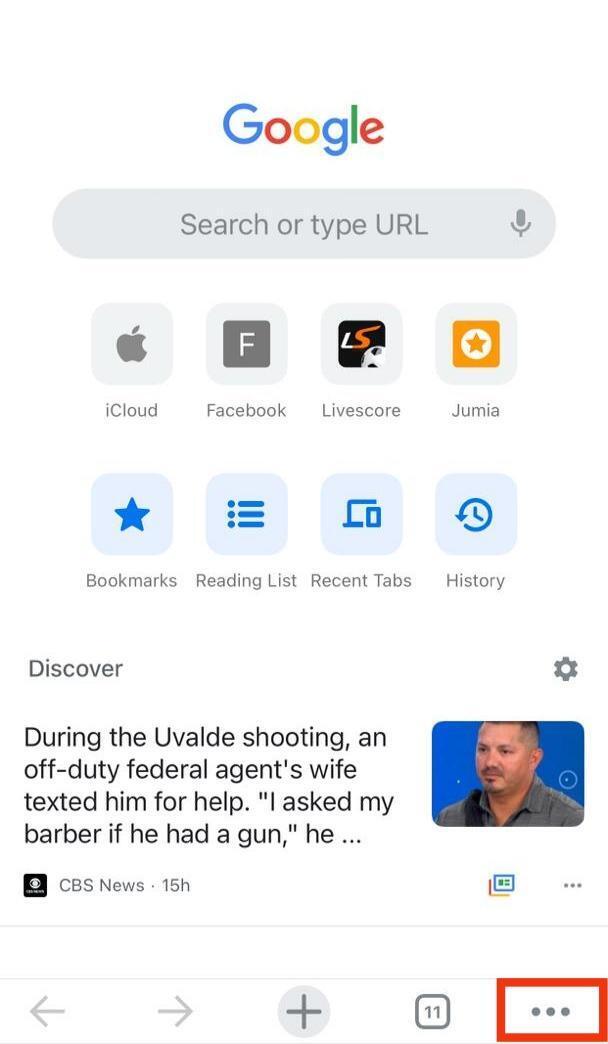This screenshot captures a Google search interface with multiple elements. At the top of the screen, the Google search bar displays a placeholder text "Type URL" and features a microphone icon for voice search. Underneath the search bar are a series of icons and text links including "Apple," "iCloud," a 'F' for "Facebook," an "LS" logo depicting a soccer ball for "LiveScore," and an orange star within a white circle on an orange square, representing "Jumia."

Beneath these, there are simpler blue icons for navigation: a blue star for "Bookmarks," a hamburger menu for "Reading List," an open laptop for "Recent Tabs," and a clock with an arrow indicating "History." These icons are presented on light blue squares with rounded corners.

The central focus of the screenshot is a snippet of a news article from CBS News. The headline reads: "During the Uvalde shooting, an off-duty federal agent's wife texted him for help. I asked my barber if he had a gun. He..." The headline is truncated with ellipses, and it's accompanied by a photo of a man on the right. The source, CBS News, is indicated by its logo on the left, and the article was published 15 hours ago. Below, there are two more logos that are not fully legible.

At the bottom of the screen, standard browser navigation icons are visible: left and right arrows, a plus sign, and a square icon with the number 11 inside it. To the right is a vertical ellipsis (hamburger-style menu) indicating more options. Notably, this screenshot highlights the hamburger-style menu with a red square for emphasis.

The clean and organized layout juxtaposes search functionalities with pertinent news updates, offering a quick, user-friendly navigation experience.